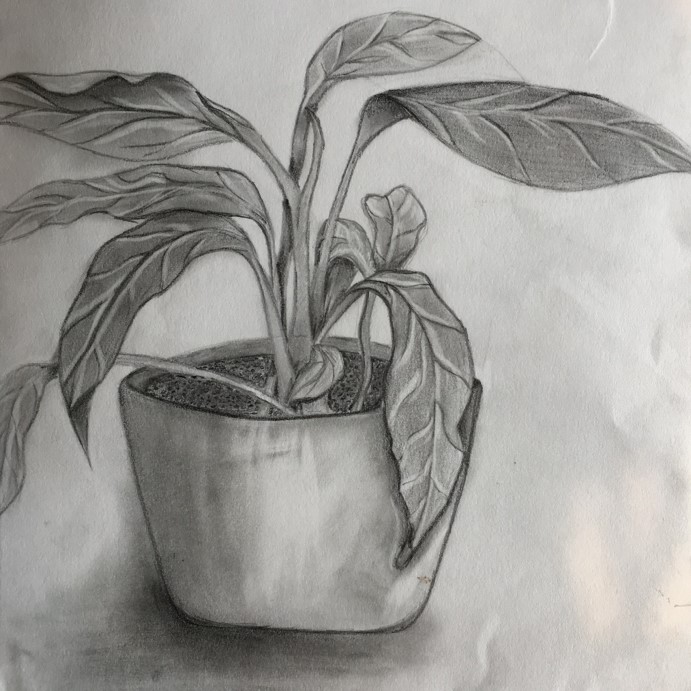The image displays a meticulously detailed pencil drawing of a potted plant on a slightly crinkled white piece of paper. The pots sits at the bottom of the composition, with its sides shaded—appearing darker towards the base to mimic a shadow. Light appears to be striking from the right side, illuminating the center of the pot and casting soft shadows toward the left.

Inside the pot, the soil is represented by a myriad of small dots, and multiple stems emerge from this base. The plant has about 10-12 leaves, displaying a range of directions and overlapping patterns. Each leaf is intricately detailed, with pronounced veins and varying degrees of shading to suggest light and shadow, contributing to a three-dimensional effect. Some leaves curl over the side of the pot, while others extend in various directions, including left, right, and upward.

Several stems branch off in different directions, some leading to leaves and others standing alone. The entire plant appears healthy and full, with leaves expertly shaded to highlight their curvature and structure. The crinkling and creases on the paper add to the texture and depth of the overall piece. Every stroke and shading technique brings out a realistic and vibrant representation of the potted plant, capturing the interplay of light and shadow.